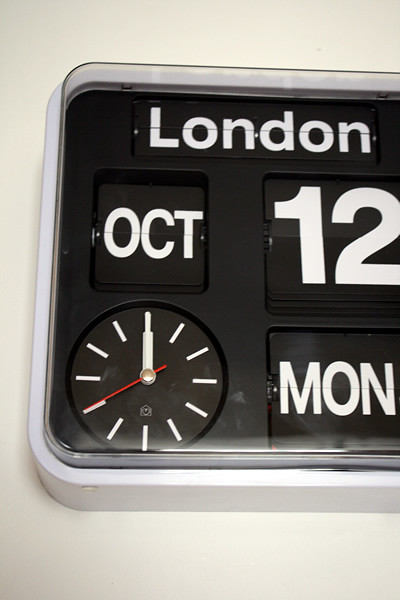This photograph captures a vintage-style clock radio against a solid black background. The main clock display features a classic flip clock design with a black background and crisp white font. In the top section of the display, the word "LON" is prominently shown, signifying the time zone or location. Below this, the date "OCT 12" appears in the same flip clock style, with "MON" indicating that it is a Monday. In the corner, there is a small, circular analog clock with black background, a white hour hand, and a red minute hand, surrounded by white dash marks representing the minutes. Covering the entire clock face is a piece of clear, glossy plastic, which reflects some ambient light, adding a touch of realistic depth to the image and emphasizing the retro aesthetic of the clock radio.